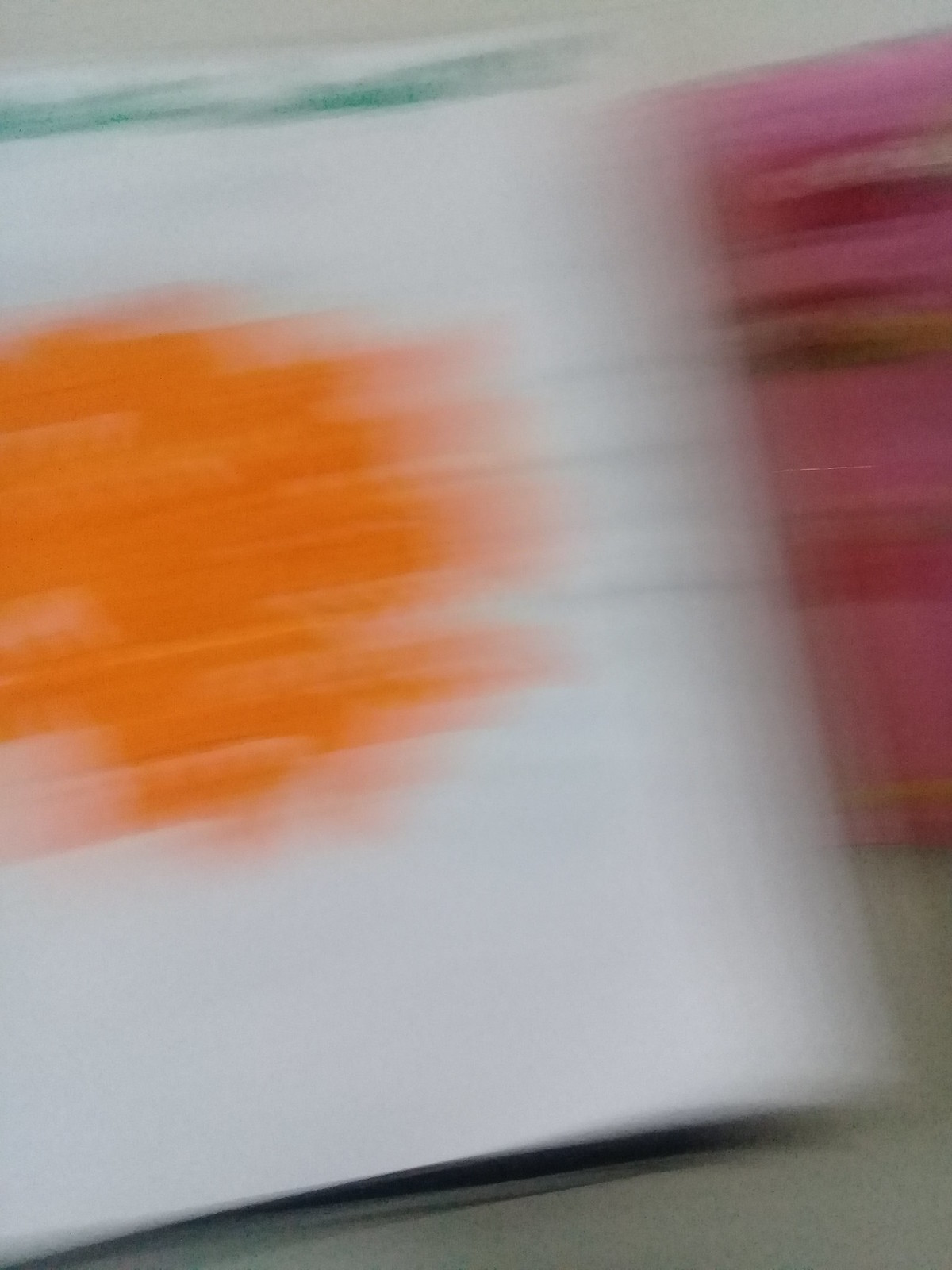This image features a very blurred photo, likely taken while the camera was in motion, resulting in lateral blurring. Central to the image is a white piece of paper or book page with an amorphous, circular orange smear in the middle, possibly created by smudging paint. A teal blue color appears at the top left of this paper, which varies in thickness and blends into the white background. This main page or book seems to cast a slight drop shadow on a gray counter surface beneath it. 

Immediately behind or next to the white page is another sheet (or book) covered with pink and red streaks that are straight across at the top and bottom. This page features a prominent dark pink stripe near the bottom and a greenish section across the middle, containing an accent with a possible brownish tinge running through it. Both pieces have a blurred, indistinct quality, with colors and shapes blending together due to the movement during the photograph.